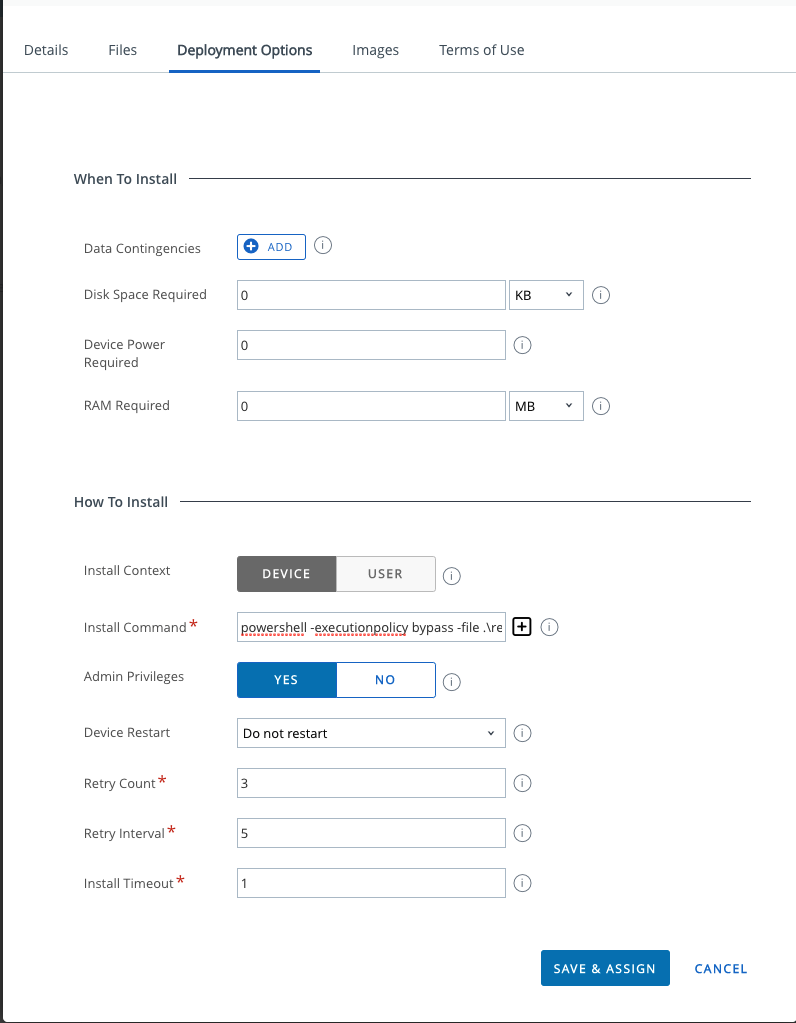Displayed on an iPad screen in portrait orientation, the screenshot centers on the "Deployment Options" tab of a software interface. The screen is predominantly white with black font text. At the top, there are five navigational tabs labeled: Details, Files, Deployment Options, Images, and Terms of Use, with the "Deployment Options" tab currently selected.

Below the active tab, the interface is segmented into two primary sections: "When to Install" and "How to Install." 

In the "When to Install" section, users can configure various parameters:
- **Data Contingencies:** Represented by an add symbol (@), indicating the option to append additional conditions.
- **Disk Space Required:** A field to input a specific numerical value.
- **Device Power Required:** Another field to enter a numerical value.
- **RAM Required:** A blank space for inputting required RAM.

The "How to Install" section outlines specific installation preferences:
- **Install Context:** Dropdown menu with options for either "device" or "user."
- **Install Command:** A text box for entering a command.
- **Admin Privileges:** Toggle options between "yes" or "no."
- **Device Restart:** A field where a specific value can be input.
- **Retry Count:** Space for a numerical entry.
- **Retry Interval:** Another field for numerical input.
- **Install Timeout:** A final field for entering numbers, specifying the allowable time for installation before it times out.

The interface appears designed to allow comprehensive customization of software deployment parameters, ensuring precise control over installation settings.